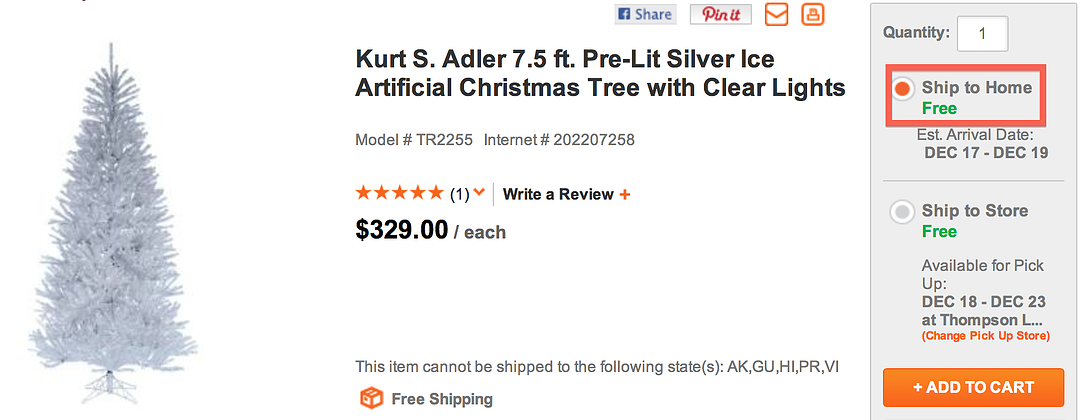Screenshot of a product search query for a Christmas tree. At the top of the page are icons for sharing via Facebook, pinning, emailing, and printing. Below those, in bold black print, is the product information: "Kurt S. Adler 7.5 FT Pre-Lit Silver Ice Artificial Christmas Tree with Clear Lights," model number TR-2255, internet number 20-220-7258. The product has a five-star rating based on one review, with an option to write a review. The price is listed as $329 each. 

A note indicates that the item cannot be shipped to Alaska (AK), Guam (GU), Hawaii (HI), Puerto Rico (PR), and the Virgin Islands (VI). Free shipping is available. On the left, a picture shows the slim, undecorated pine tree standing on a wire stand. 

On the right, the purchase options are displayed. Quantity is set to one, with the chosen shipping method being "Ship to Home Free," with an estimated arrival date of December 17th through December 19th. Another option, "Ship to Store Free," is available for pickup between December 18th and December 23rd at Thompson L, with a clickable link to change the pickup store. Finally, there is a rectangle button labeled "Add to Cart."